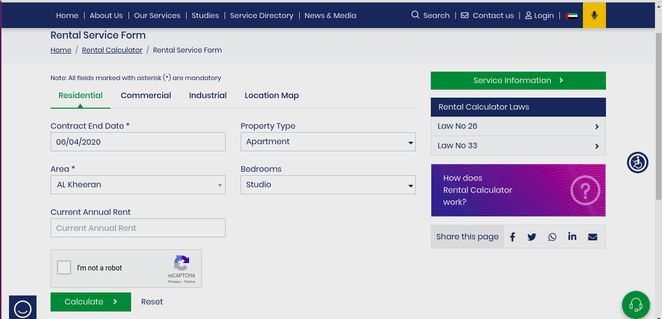This detailed caption accompanies a cropped screenshot of a website's rental service form set against a light gray background. At the top left, the heading "Rental Service Form" is prominently displayed. Below this heading, there are navigation links labeled "Home," "Rental Calculator," and "Rental Service Form."

Further down, a note reads: "All fields marked with an asterisk are mandatory." The form is divided into three categories: Residential, Commercial, and Industrial, with Commercial being the selected category, highlighted in green with a green horizontal line underneath it. The text is small and blue for all categories except the selected one.

To the right of these categories, there is a location map displayed. Underneath the selected category (Commercial), the form includes text boxes for "Contract End Date," "Area," and "Current Annual Rent." To the right of these text boxes, there are two dropdown menus: one for apartment type and another for the number of bedrooms.

At the bottom left of the form, there is a captcha feature that includes a checkbox labeled "I’m not a robot." Directly below this, there is a green button labeled "Calculate" with an arrow pointing to the left, and to its right, a smaller gray "Reset" button.

On the far left side of the page, there is a green button labeled "Service Information," followed by a section labeled "Rental Calculator" and a purple box with the text "How Does Rental Calculator Work?" Underneath these, there is a gray box that encourages users to "Share This Page," accompanied by icons for Facebook, Twitter, Telephone, Indeed, and an envelope to facilitate sharing via various platforms.

In the bottom right corner, there is a green circle with a headset icon, and towards the center right, there is a blue handicap accessibility icon.